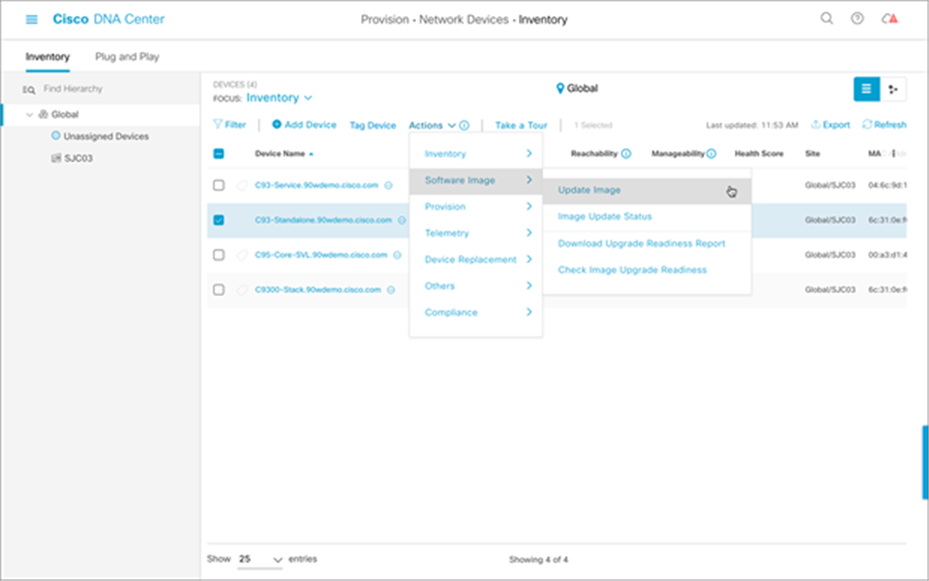The image depicts a white background with a light gray horizontal line running across the top. In the upper left corner, a small turquoise-colored square bears the words "Cisco DNA Center." To the right of this, black text reads "Provision Network Devices and Inventory." In the upper right corner, there are three icons: a magnifying glass, a circle with a question mark, and a red triangle.

Below this section, a sidebar is visible. At the top, the sidebar title reads "Inventory Plug-and-Play." Beneath this, a search bar labeled "Find Hierarchy" is positioned. Below the search bar, the word "Global" is displayed, and when clicked, it expands to reveal two files named "Unassigned Devices" and "SJC 03."

The image combines navigational elements with functional icons, effectively organizing the layout for network device management within the Cisco DNA Center interface.